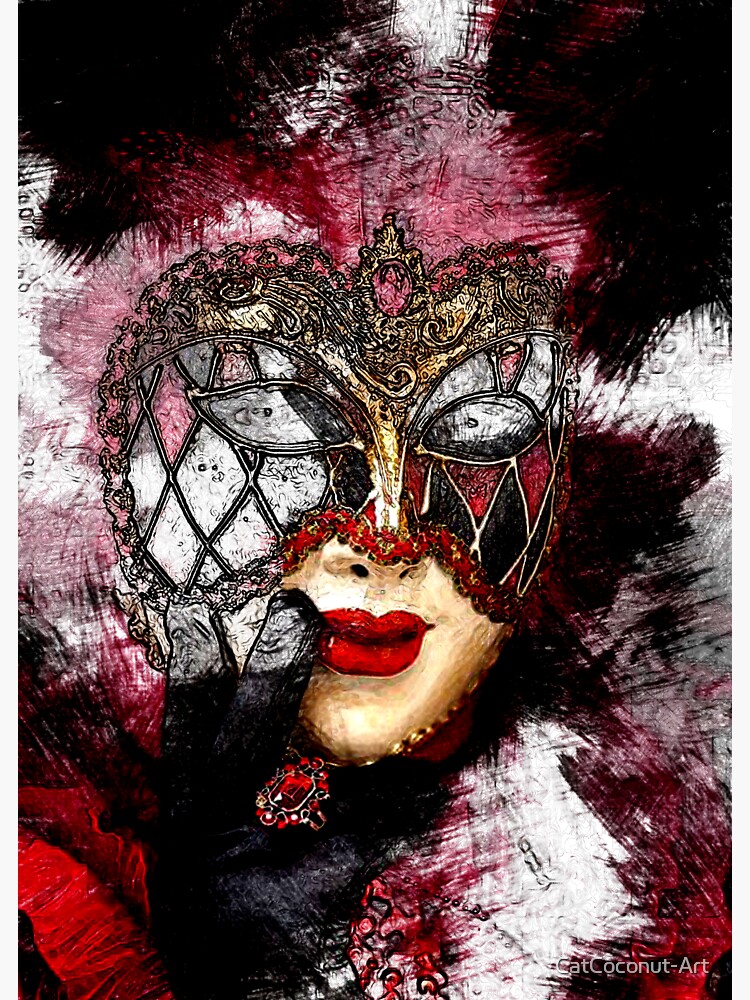This is a fantastical, artistic rendering by Cat Coconut-Art, presented in portrait orientation. The focal point is a woman dressed in a vibrant and elaborate jester-like costume. Her face, painted in a stark white, is adorned with bright red lipstick and partially covered by a highly ornate Baroque mask. This mask features a bronze and goldish hue, highlighting her facial features. Her eyes, striking and white with tiny pupils, peer through the mask's eye coverings, which are patterned in black and red diamonds over the left eye and white and pink diamonds over the right eye. Emerging from the back are bright red and white flowers that add to her jester appearance. She wears a black glove on her hand, which is tucked thoughtfully under her chin, showcasing a large red ring on her ring finger. The attire is a blend of red, white, and black, marked by abstract patterns and textures created through visible brush strokes, adding depth and character to the costume. A red brooch adorns her neck, completing her enigmatic and elaborate masquerade look.